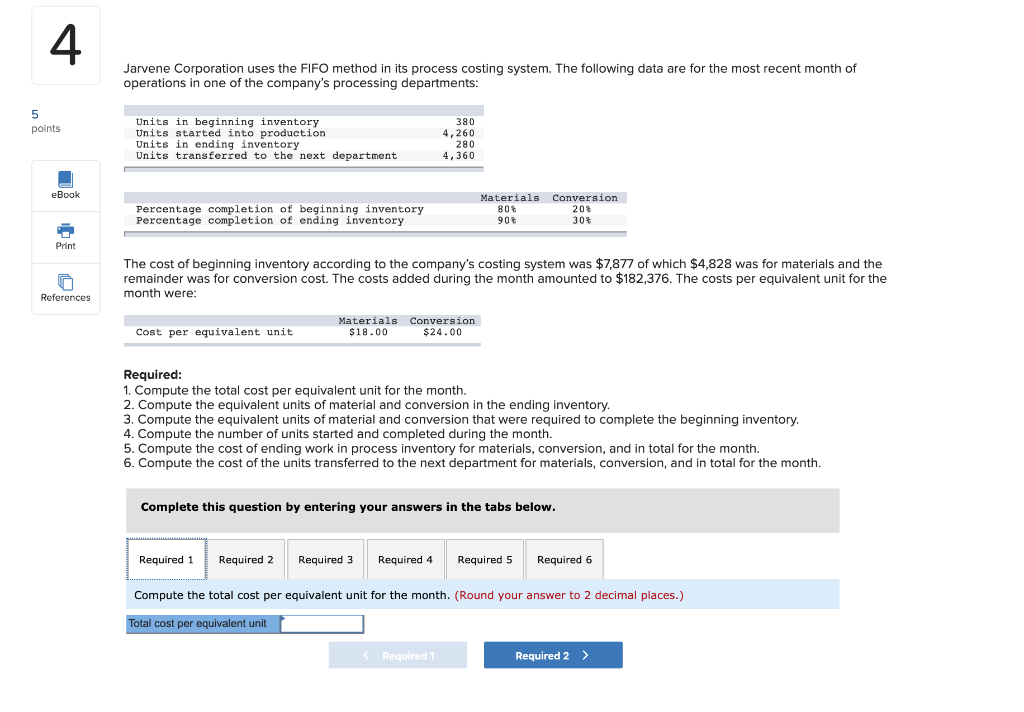The image portrays an antiquated website, presented in the classic Times New Roman font, reminiscent of early 2000s web design. The site features basic text and minimalistic elements, with a noticeably simple layout. In the top left corner, there is a small box containing the number '4', below which it states 'five points'. Further down, the menu options include 'ebook' accompanied by a small book icon, 'print', and 'references' with additional page icons, all contributing to its vintage appeal.

Dominating the page is a section of text, presumably in approximately 10-point Times New Roman, detailing a process cost accounting scenario for Jarveen Corporation. The text states: "Jarveen Corporation uses the FIFO method and its process costing system. The following data are for the most recent month of operations in one of the company's processing departments." This introduction is followed by a structured table with alternating gray and white rows, listing:

- Units in beginning inventory: 380
- Units started into production: 4,260
- Units in ending inventory: 280
- Units transferred to the next department: 4,360

Another table provides percentages for the completion of beginning inventory materials and conversion. The cost details are elaborated, noting that the beginning inventory cost was $7,877, with $4,820 allocated to materials and the remainder to conversion costs. Additionally, the costs added during the month amount to $182,376.

Towards the bottom of the page, there is a 'Required' section listing six items, each associated with a small clickable square. These likely link to further details or related tasks. Below this, navigation options suggest the ability to proceed to subsequent pages. The overall design and content suggest instructional or educational material, characteristic of older, straightforward web interfaces.